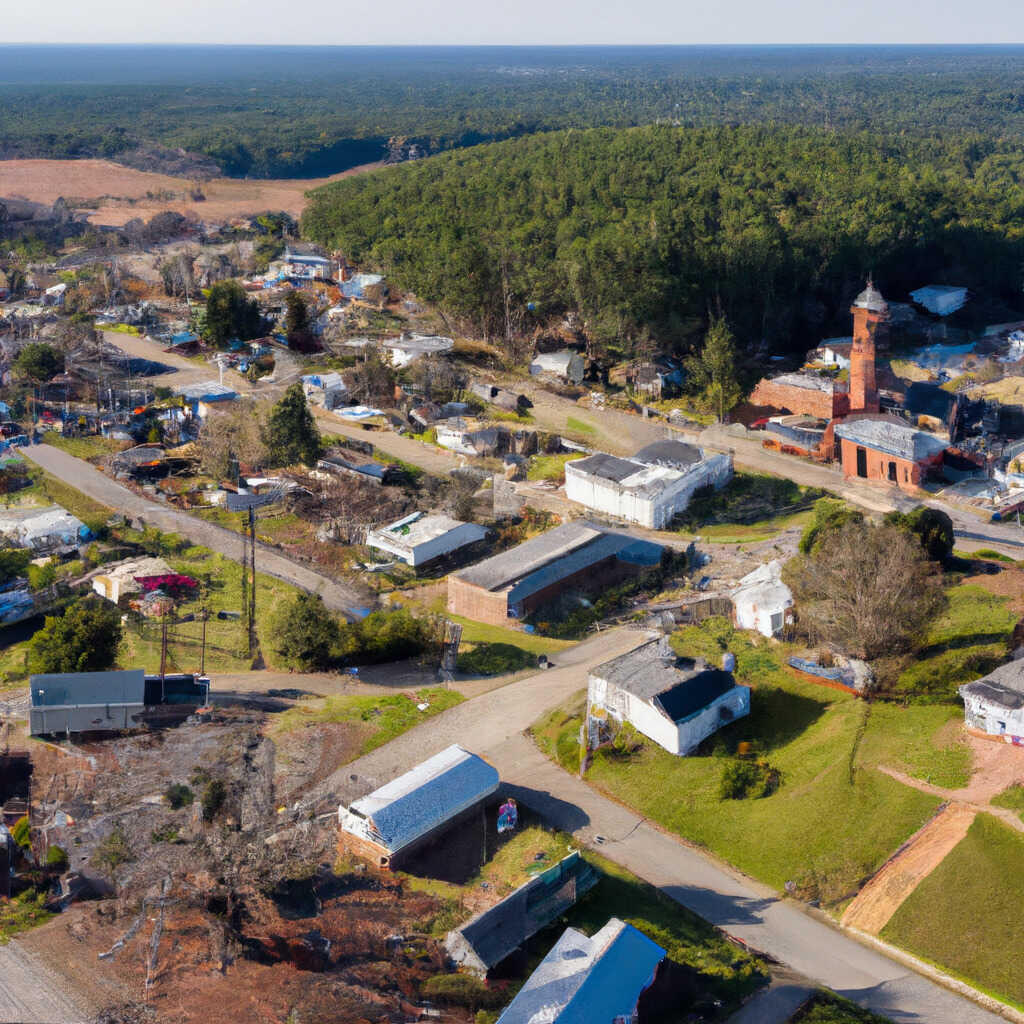This is an aerial photo of a seemingly abandoned city, reminiscent of an old mining town, featuring a maze of narrow streets lined with numerous buildings in various states of disrepair. The most prominent structure is a brick-colored building with a tall tower and circular roof, positioned toward the middle right edge of the image, surrounded by two smaller brick-colored buildings. Many structures have blue tarps on their roofs, suggesting recent damage, possibly from a natural disaster. Scattered trucks and industrial equipment are visible, indicating a formerly active site now devoid of life. Green patches of grass and a few trees stand out amidst the decay. In stark contrast, the background reveals a dense forest extending to the horizon under a hazy white sky. Evidence of a past flood is present, as indicated by muddy, barren areas, further emphasizing the town's abandonment and the desolate atmosphere.